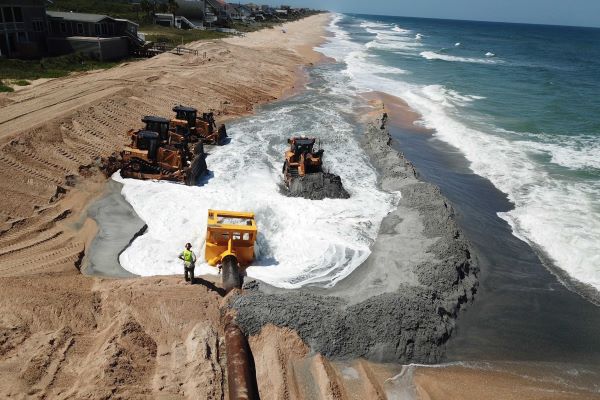An aerial photograph captures a bustling coastline construction site where multiple excavators are actively piling sand to create a barrier between the ocean and the shore. The vibrant blue waves crash against the sandy beach to the right, their white foam encroaching onto the construction zone. Dominating the center of the image, the site is partially submerged in water, possibly due to tidal influences, complicating the workers' task. A key feature in the scene is a large pipe, likely intended for drainage, extending from the waterlogged area into the sand. A solitary figure, identifiable by his yellow safety vest and helmet, stands attentively next to one of the yellow excavators, possibly assessing the situation. The backdrop reveals a gentle rise of sand to the left, with houses visible in the distant landscape, underlining the human impact on this coastal environment.